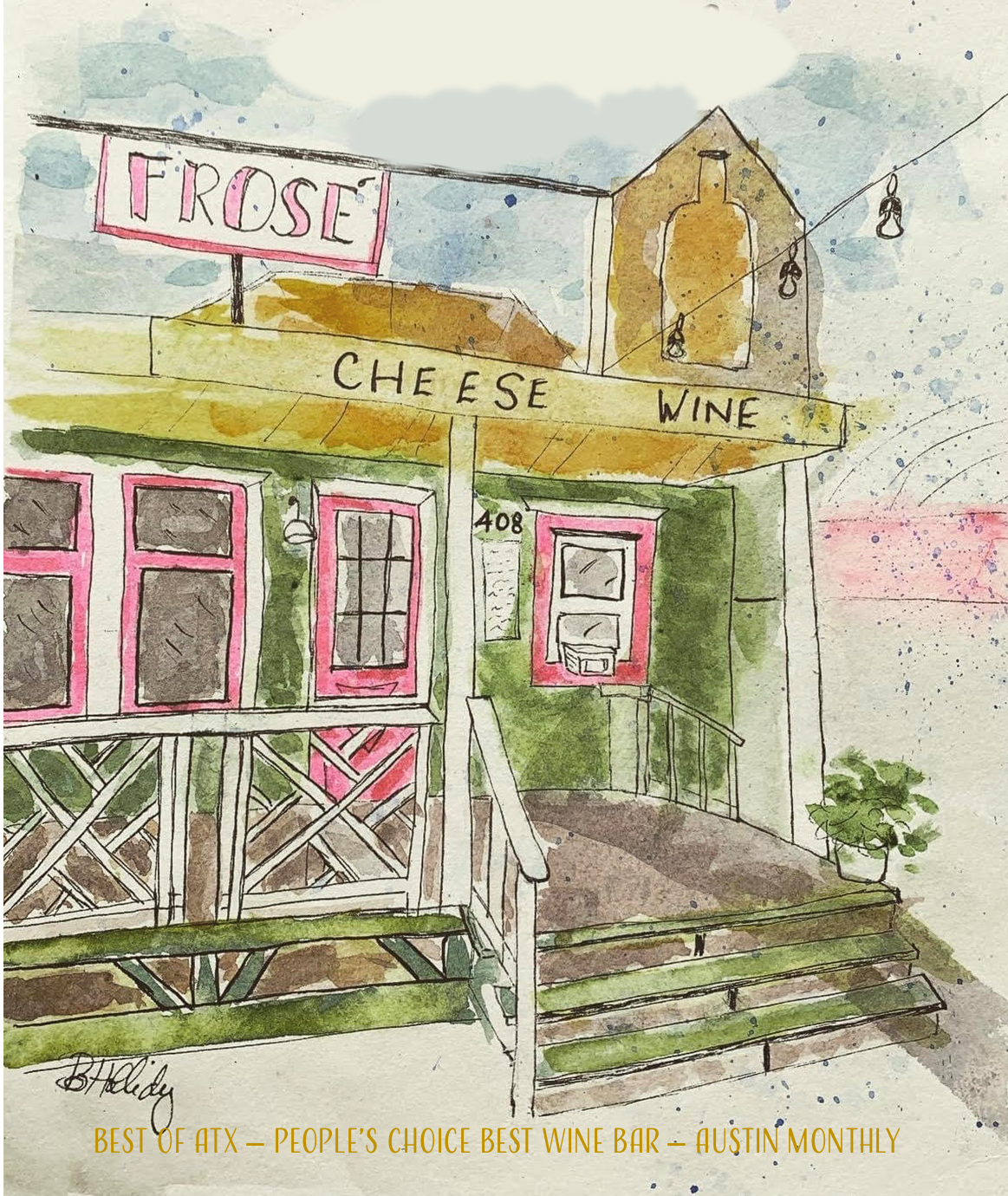This image is a vibrant, cartoonish watercolor painting of a charming wine and cheese shop. The building is distinguished by its green siding and a whimsical, covered porch featuring a white banister and green steps partially covered in concrete. The porch is accented with pink window sills and a pink front door, prominently displaying the black house number "408" next to an exterior light. 

Atop the porch roof, a sign in bold pink letters spells out "Frosé" (F-R-O-S-E), indicating frozen wine, and a drawing of a wine bottle is displayed prominently. Above the main roofline, another sign reads "Cheese and Wine," emphasizing the shop's offerings. 

Strung above the shop's entrance is a festive string of lights, adding to the playful atmosphere. Potted green plants adorn the three steps leading to the porch, enhancing its inviting ambiance. In the background, the sky is depicted in shades of gray, blue, and white, providing a soft, tranquil backdrop to the lively portrayal of the building. 

Across the bottom of the image, in uppercase dark yellow text, the accolades "Best of ATX - People's Choice Best Wine Bar - Austin Monthly" are displayed, suggesting this artwork might feature in promotional material or a review. The piece is signed by the artist, "Bee Holiday," in a scrawled black signature.